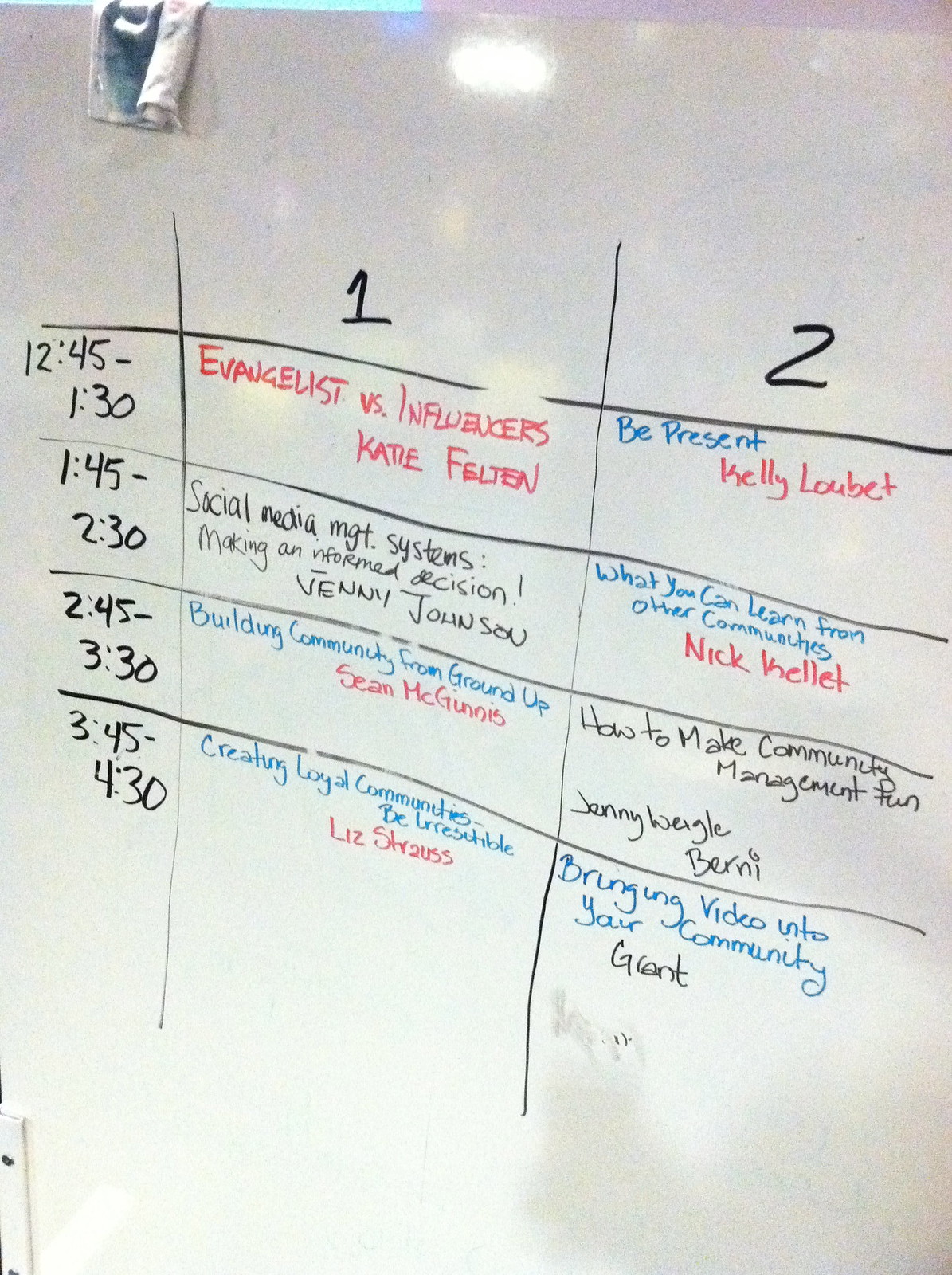The photograph depicts an off-white rectangular whiteboard, situated indoors, reflecting an overhead light at the top center. The board showcases a detailed schedule of professional development sessions, organized into three columns in black, red, and blue marker. The schedule spans four time slots from 12:45 PM to 4:30 PM, with the leftmost column listing these times. The middle column, labeled "1," and the rightmost column, labeled "2," each feature distinct session titles and speaker names for each time slot:

- **12:45 PM to 1:30 PM:**
  - Column 1: "Evangelist vs. Influencers," Katie Felton
  - Column 2: "Be Present," Kelly Loubet

- **1:45 PM to 2:30 PM:**
  - Column 1: "Social Media Management Systems: Making an Informed Decision," Jenny Johnson
  - Column 2: "What You Can Learn from Other Communities," Nick Kellett

- **2:45 PM to 3:30 PM:**
  - Column 1: "Building Community from the Ground Up," Sean McGinnis
  - Column 2: "How to Make Community Management Fun," Jenny Weigel-Bernie

- **3:45 PM to 4:30 PM:**
  - Column 1: "Creating Loyal Communities: Be Irresistible," Liz Strauss
  - Column 2: "Bringing Video into Your Community," Grant

The varied handwriting and marker colors imply that the presenters themselves might have written their respective sessions on the whiteboard. The organized schedule offers attendees a selection of eight sessions, each designed to enhance skills and knowledge in community building and social media.